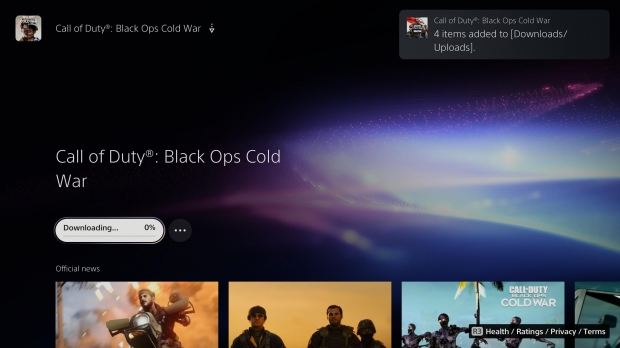This screenshot features a predominantly black background with a notable burst of muted, blended colors on the right side, slightly above center. The colors—maroon, dark blue, light blue, light green, gray, and purple—form an abstract shape resembling an oval with a curved-in triangle underneath. In the upper left corner, there is a white square containing the head of a person. To the right of this square, the text "Call of Duty: Black Ops Cold War" is prominently displayed in white, accompanied by a gray downward-pointing arrow. Midway down the left side, the phrase "Call of Duty®: Black Ops Cold War" appears in gray text. Below this, about two lines down, a long white oval contains the black text "Downloading" on the left and "0%" on the right, with three white dots situated just outside to the right of the oval. At the bottom, the screenshot includes part of a visual gallery: there is a narrow blank space followed by three visible pictures, with the left edge of a fourth picture faintly visible at the far right.